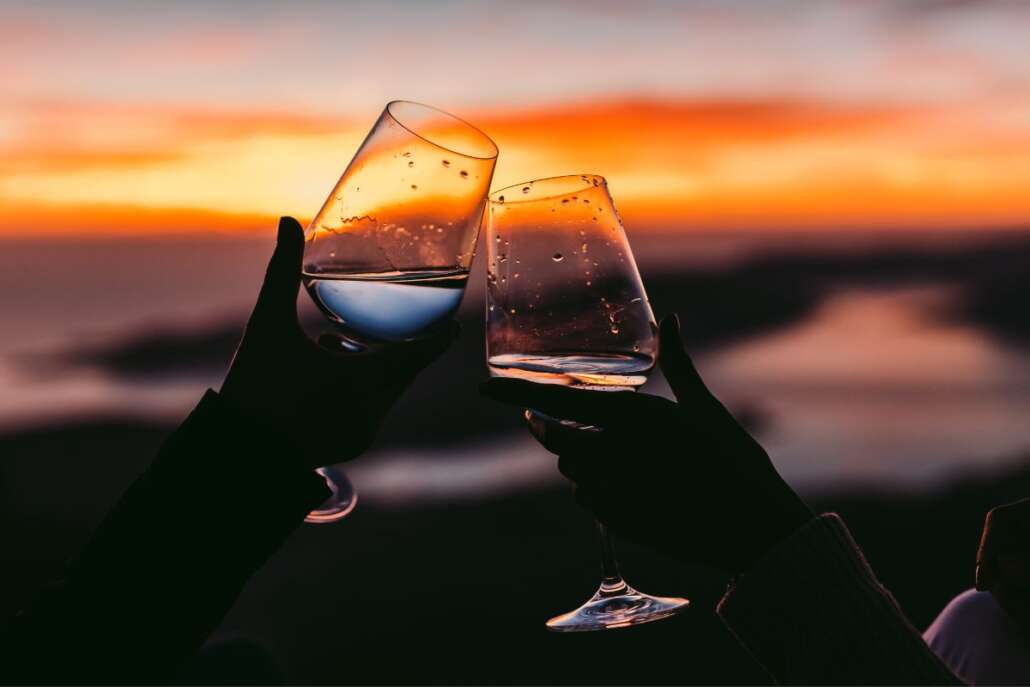This evocative and artistic image captures two individuals in a celebratory moment as they clink their clear wine glasses, which contain a light, possibly clear liquid such as champagne, white wine, or water. The glasses are adorned with droplets, suggesting the coolness of the liquid inside. The scene is set against a striking backdrop of a sunset, where hues of orange, pink, and purple merge seamlessly, casting a purple haze over the lower part of the image. The dusk light illuminates the partly silhouetted hands holding the glasses, adding to the dramatic effect. The fading light creates a soft glow in the sky, blending yellow and orange light through gauzy clouds. The setting hints at an outdoor, perhaps beachside location, with gentle waves pooling on the right side of the image, further enhancing the tranquil and celebratory ambiance.